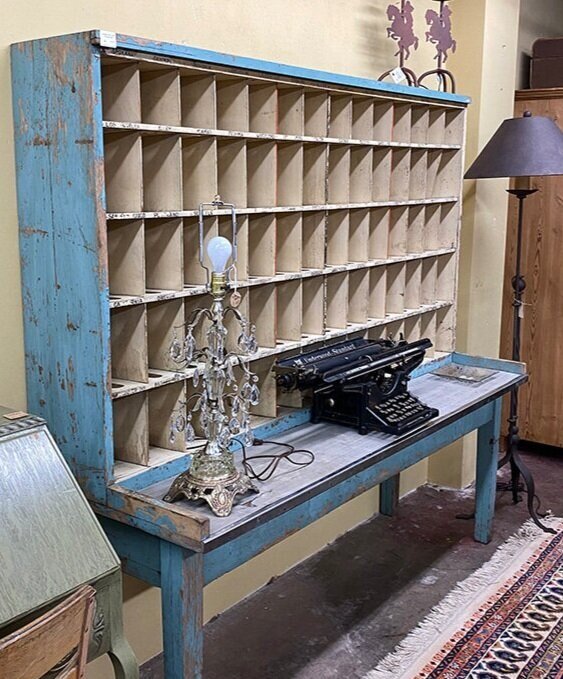The image captures an antique room with a worn, brown wooden floor that urgently needs refinishing. The floor partially reveals the fringed edge of a patterned rug incorporating red, black, white, and blue tones. Positioned against a beige wall, the primary focus is a distressed shabby chic style table painted in a fading bright teal blue, indicative of its age and extensive use. Rising from the back of the table are five rows of wooden mail sorting slots from an older era, approximately fifteen to eighteen cubbies running across each row, all currently empty. 

On the tabletop sits a variety of antiquities: a highly ornate brass lamp adorned with hanging crystals, although missing its lampshade and connected to an unplugged cord with a single white light bulb evident; and directly beside it, a strikingly black typewriter from the 1920s arranged as if for display. To the extreme right of the table, a dark-colored floor lamp with three legs stands tall, its tan lampshade reaching the height of the mail slots. 

Another old student desk with a gray metal frame and a wooden chair typical of public schools from decades ago peeks in from the left side of the image. There are indications of additional raw iron ironwork present, possibly decorative items, alongside a small tray on the table adding to the vintage ambiance.